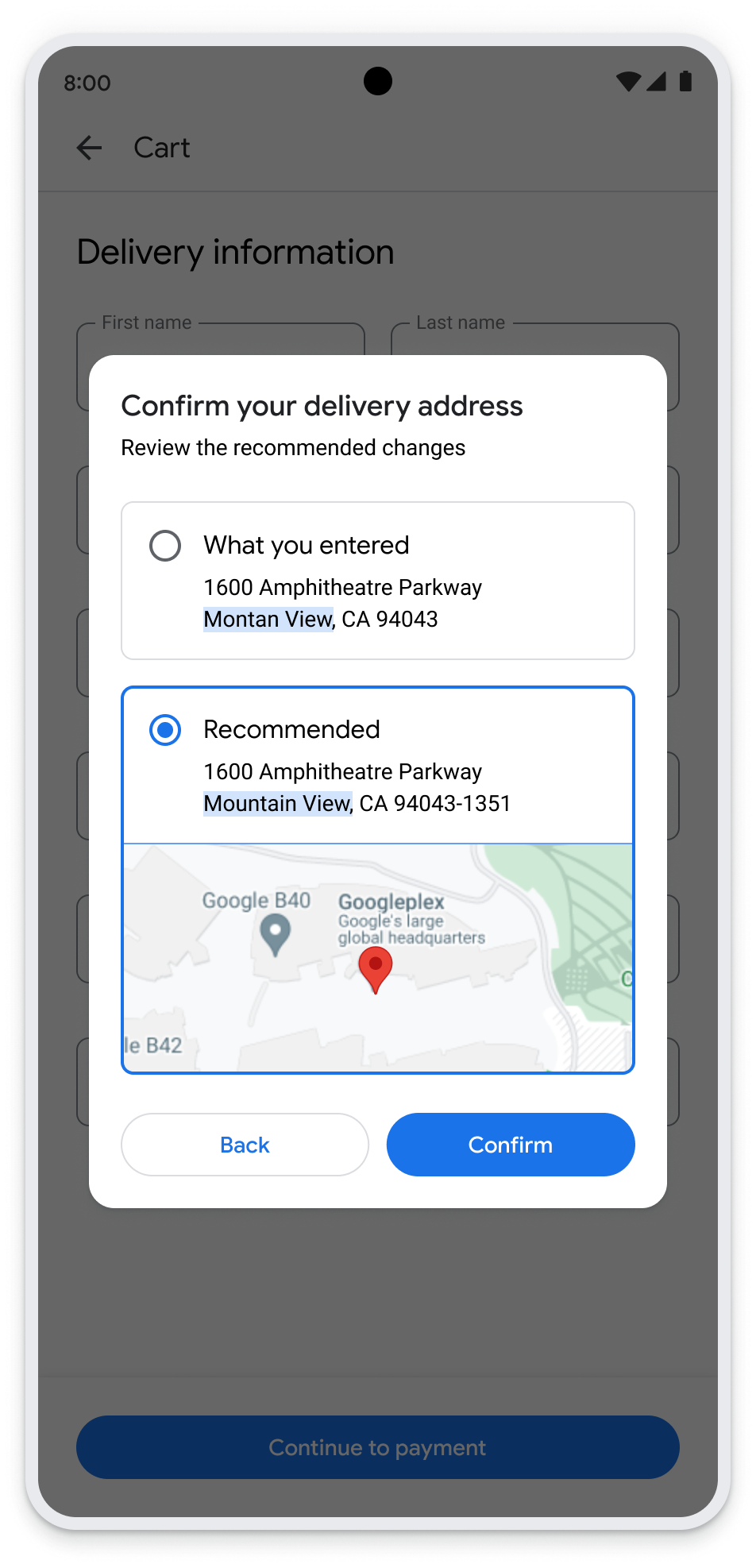This image appears to be a screenshot of a simulated phone screen displaying a delivery address confirmation page on an e-commerce platform. 

The background of the screen is a faintly grayed-out white, creating a backdrop for the interface elements. 

At the very top, there is a header that reads "8," accompanied by a "Cart" label with a back arrow next to it. To the right, the status bar shows a Wi-Fi icon, a battery icon, and a signal strength icon. 

The main content area is blurred, likely due to an overlay pop-up, but some information is still discernible. It includes a section labeled "Delivery Information" in black text, with two visible black boxes for "First Name" and "Last Name."

Dominating the central part of the screen, a white pop-up lays over the blurred background. The top of the pop-up features black text reading "Confirm your delivery address. Review the recommended changes." Below this, there's a gray circle next to the text. The text "What you entered: 1600 Amphitheater Parkway, Mountain View, California 94043" is displayed in black.

Directly beneath, a recommended address is framed with a blue border and a blue-dotted circle indicating selection. The recommended address reads "1600 Amphitheater Parkway, Mountain View, California 94043-1351."

Integrated within the pop-up is a miniature view of Google Maps, featuring a gray pin and a red pin. Accompanying this map, labels identify the location as "Google B40, Googleplex, Google's large global headquarters."

At the bottom of the grayed-out background, there is a blue and white button that reads "Continue to Payment." The pop-up also includes two buttons: a white "Back" button outlined in blue, and a blue "Confirm" button with white text.

Overall, the image is a detailed capture of a delivery confirmation step within a mobile shopping interface, complete with precise location confirmation and the option to proceed to the next stage of the checkout process.